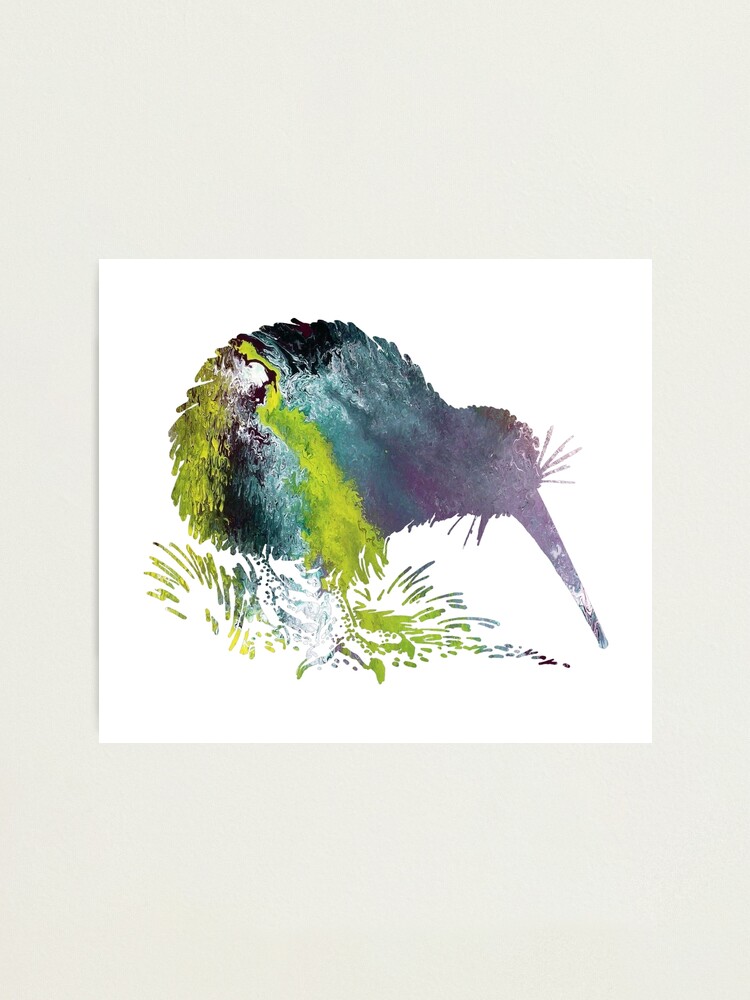This image features a watercolor painting of a kiwi bird set on a white square canvas, which appears to be mounted on a light gray, almost beige, vertically oriented rectangular background. The kiwi bird, depicted in profile and facing to the right, is characterized by its long, sharp beak and colorful, metallic-like plumage. The bird's head is a faded purple, transitioning through blues and greens towards its back feathers which include dark green and near-black hues. The painting style is somewhat abstract, focusing on smudges and blends of these colors rather than intricate details. The kiwi stands amidst blades of grass, with its speckled feet visible beneath its body, adding an element of the natural environment to the composition.